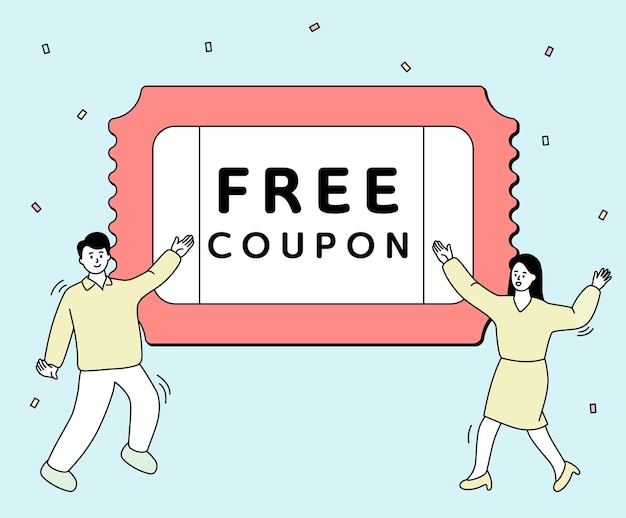In this graphic image, two cartoon-style figures, a man on the left and a woman on the right, are depicted against a light turquoise blue background. The man has black hair and is pointing towards a centrally placed ticket, resembling an old-school carnival ticket with an orange-red border. The ticket bears the bold, uppercase text “FREE COUPON” in black. The woman figure also has black hair, is dressed in a green long-sleeved V-neck shirt paired with a green skirt and green high heels. The man is similarly clad in a green shirt and lighter green shoes. Both figures feature simple facial expressions with stick figure-like eyes, noses, and mouths, but their bodies are more rounded with visible arms and legs. Confetti in various shapes and colors, such as brown and yellow squares, is scattered around the scene, adding a festive touch to the minimalistic yet charming illustration.